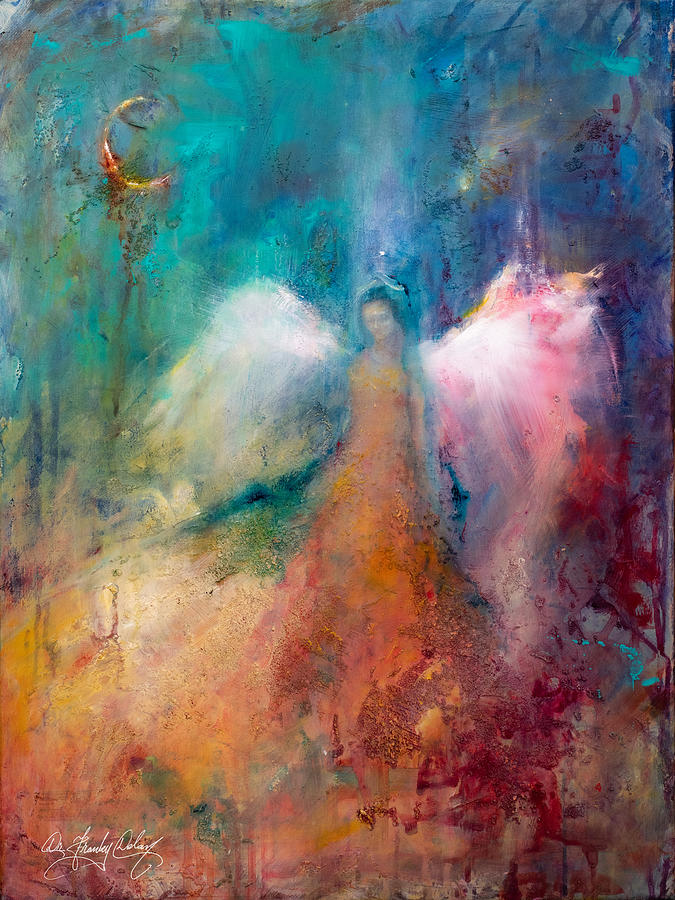This detailed oil painting features a somewhat abstract representation of a female angel at its center, predominantly dressed in a flowing orange dress with hints of yellow and brown hues. Her long dark hair and slightly blurred white wings add an ethereal quality as they blend into the multi-colored, indistinct background filled with vibrant splotches of red, green, and tan. The backdrop lacks a definitive structure, enhancing the painting’s abstract nature, yet it provides a surreal, dreamlike landscape where the ground beneath the angel appears to be a hill of varied colors including light tan, orange, green, and red. In the upper left-hand corner, a crescent moon or possibly a solar eclipse graces a bluish-teal sky. Despite these blurred and blended elements, the painting exudes a sense of mysticism and vivid coloration, indicative of an oil medium. The piece is signed in white cursive in the lower left corner, although the artist’s name remains indistinguishable even under closer inspection.